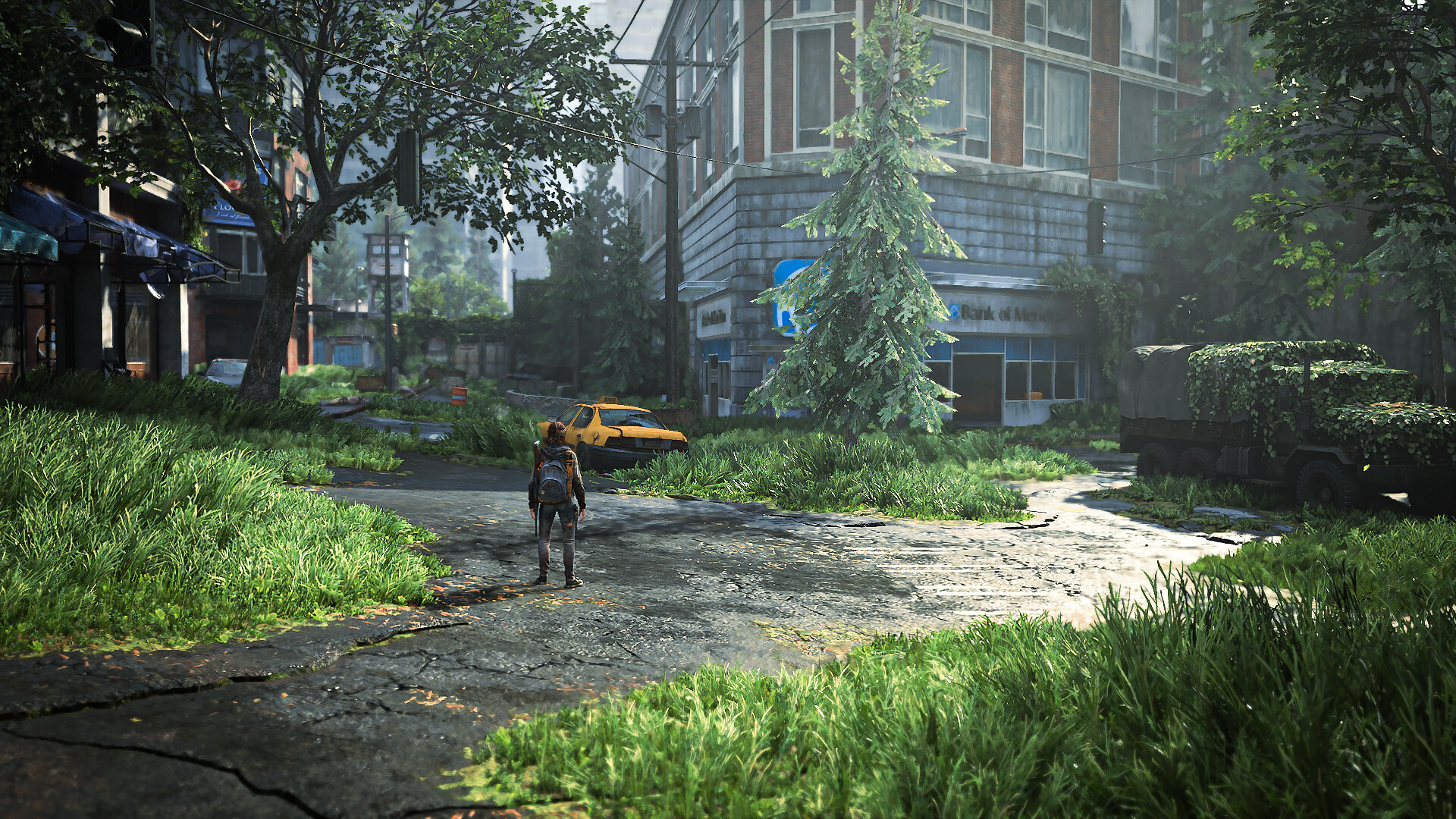This image appears to be a still from a video game, rendered with computer-generated graphics. The scene depicts a desolate city overtaken by nature, with overgrown vegetation encroaching on buildings and vehicles. On the right side of the image, a military truck is almost obscured by greenery, indicating long-term neglect. The background features several abandoned cars and miscellaneous debris, enhancing the sense of abandonment and decay. At the image's center stands a woman, identifiable by her shoulder-length hair tied back in a simple style. She is equipped with a backpack and wears tight pants, sturdy boots, and a leather jacket, suggesting she is prepared for travel or survival. The woman gazes away from the camera, focusing on an empty yellow car ahead of her. The setting appears to be a small city center, now eerily silent and devoid of life. There is no text in the image.